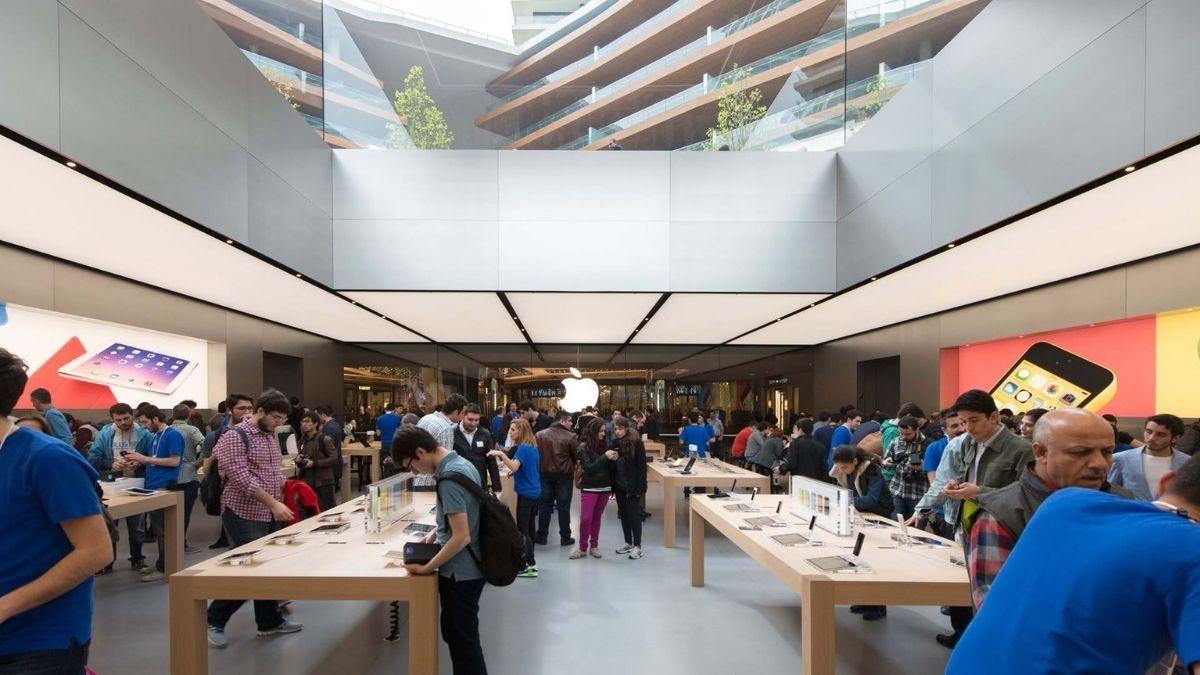In this bustling Apple store, the image captures the interior with around 50 to 60 people scattered throughout. Shoppers of various age groups are seen socializing and examining products placed on tan wooden desks. These desks, characterized by their simple design with four legs and flat rectangular surfaces, are laden with electronics. The store’s modern and futuristic aesthetic is highlighted by the prominent white Apple logo displayed at the far end. 

The architecture includes white undersides of the walls that transition into gray as they rise, complemented by a matching gray floor. To the left and right, signs indicate the cell phone section. Adding to the sophisticated ambiance, the ceiling is made of glass, providing a view of the exterior. Beyond the ceiling, there’s a glimpse of a tall building with distinct brown vertical rows and a touch of greenery from a tree peeking through. The combination of sleek design, diverse clientele, and meticulously arranged products creates a dynamic snapshot of this Apple store environment.